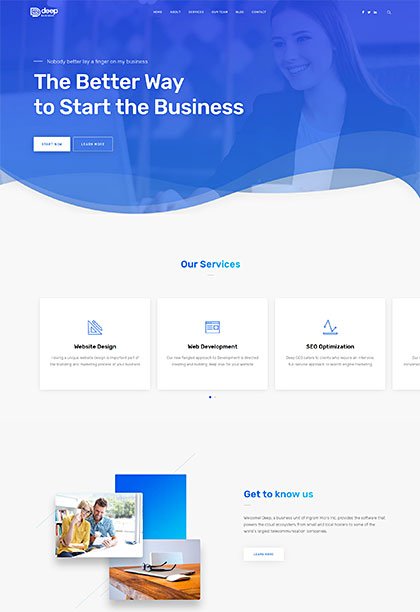This is a detailed, cleaned-up caption for the image described:

"This is a cropped, full-page screenshot of a website, with the entire top bar removed. At the top of the image, the background features a photo of a woman working behind a computer, overlaid with a blue filter. In the top right corner of the image, there are three vertical dots followed by a very small blue button. At the top center, a list of categories is displayed vertically in small white letters. The logo is positioned on the far left.

Overlaying the photo, a large white slogan reads, 'The Better Way to Start the Business.' Below this slogan, two buttons are positioned side by side. The button on the left is white with blue text, and the one directly to its right is blue with white text.

The lower part of the screenshot has a white background with the heading 'Our Services' centered in small letters. Below this heading, there are three fully visible large white squares, each with an icon in the center and a description beneath it. The edge of a fourth square is partially visible, indicating the user can scroll through additional service options. However, due to the crop, the scroll bars or additional boxes are not visible.

At the bottom of the image, the section titled 'Get to Know Us' features a collage of three pictures on the left. To the right of the collage, there is a description and a white button with blue text. Due to the cropped and minimized nature of the website photo, the smaller text in this section is not legible."